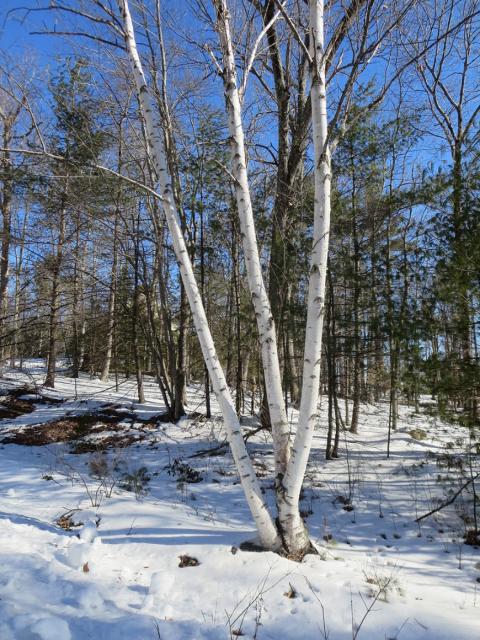The image portrays a serene winter scene set in the middle of a forest, characterized by a blue sky that suggests daytime with the sun shining brightly. Dominating the foreground is a striking birch tree with white bark, notable for its three distinct trunks emerging from a single root, forming a unique triad. Some knots in the bark are black, adding contrast. The birch is devoid of leaves, as are the multitude of small trees that populate the background, their bare branches stretching towards the sky.

Surrounding the birch tree and scattered throughout the scene are sparse patches of green grass and small berry bushes, their starkness accentuated by the snow covering the forest floor. The snow depth appears to be about one or two inches, with patches of brown dirt sporadically peeking through, particularly in the left-middle portion of the image. The evergreen trees, cloaked in green, stand towards the back, providing a vivid backdrop to the mostly gray, brown, and white hues of the wintery forest landscape.